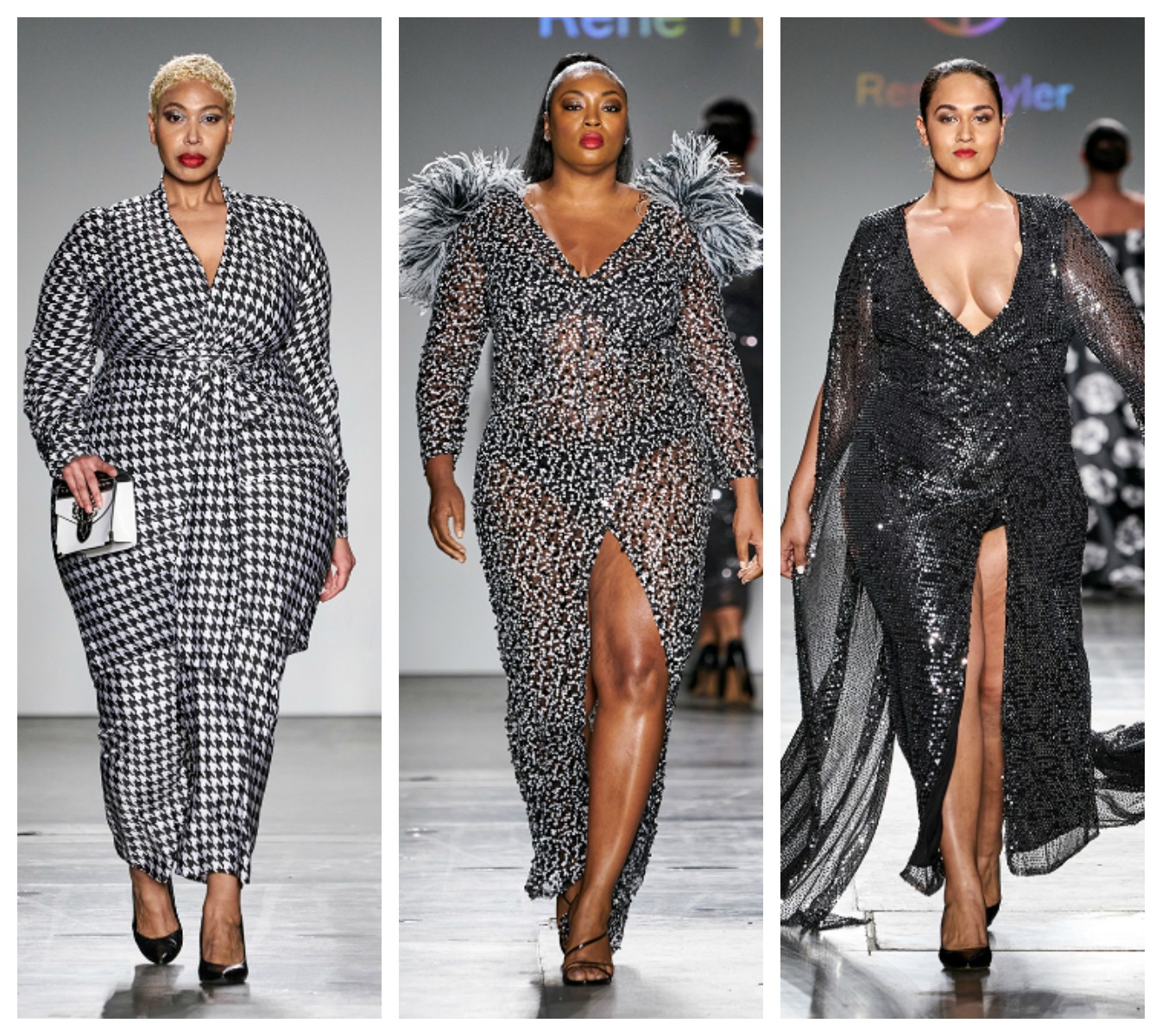In this striking image, three plus-size models are showcased on a fashion runway, set against a light gray background with a black floor, divided into three vertical rectangles by white lines.

On the left, a black model with short, slightly curly blonde hair and red lipstick wears a chic, houndstooth-patterned outfit—a blend of gray, black, and white—with a bow at the waist. She accentuates her look with a white clutch and black high heels, embodying a balance between casual and office wear as she strides confidently.

The central figure, a black model with long brown hair cascading behind her shoulders, dons an elegant black and white dress featuring a V-neckline. The dress, adorned with a floral pattern and fluffy ruffles on the shoulders, has a slit above the knee on the left leg, revealing fashionable sandals. Both her demeanor and attire exude sophistication.

On the right, another black model with short dark hair and red lipstick showcases a daring, low-cut black dress. The dress, semi-transparent on the upper arms and intricate with mesh details, forms a circular V below the chest, subtly revealing cleavage. The ensemble, complete with a high slit on the upper thigh, includes a train-like extension below her right arm, adding dramatic flair as she walks.

All three models, serious-faced and poised, traverse a gray platform, epitomizing bold elegance in this high-fashion scene.